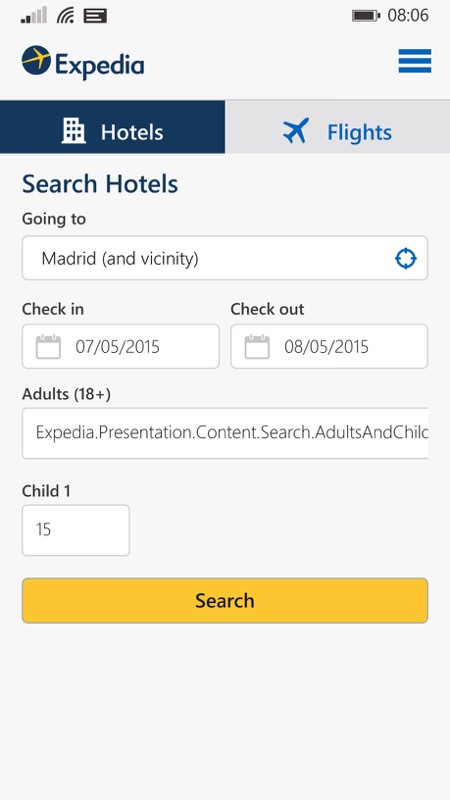This image is a detailed screenshot from an Expedia page for searching hotels. At the top left corner, the Expedia logo is prominently displayed, consisting of the word "Expedia" in dark blue and a dark blue circle icon with a yellow plane flying across it. To the right of the logo, there is a menu icon depicted as three horizontal bars in a lighter shade of blue.

Beneath the logo and menu icon, there are two primary navigation tabs. The left tab, representing "Hotels," is a solid dark blue and features white text that reads "Hotels" alongside a white building icon. The right tab, which is light gray, signifies "Flights" and displays blue text reading "Flights" along with a plane icon.

Directly below these tabs, the interface instructs users to "Search hotels" written in dark blue text. The first step in the search process indicates the destination with the phrase "Going to" and a selected field that specifies "Madrid (and vicinity)."

Following the destination input, the screen provides fields for selecting check-in and check-out dates. The "Check-in" option is positioned on the left, while "Check-out" is on the right, both accompanied by a date selector tool.

Further down, the booking form prompts users to specify the number of adults with the label "Adults, 18+." Below the adult selection, there is a field for specifying the number of children, labeled "Child 1," which currently shows "15" within the input box.